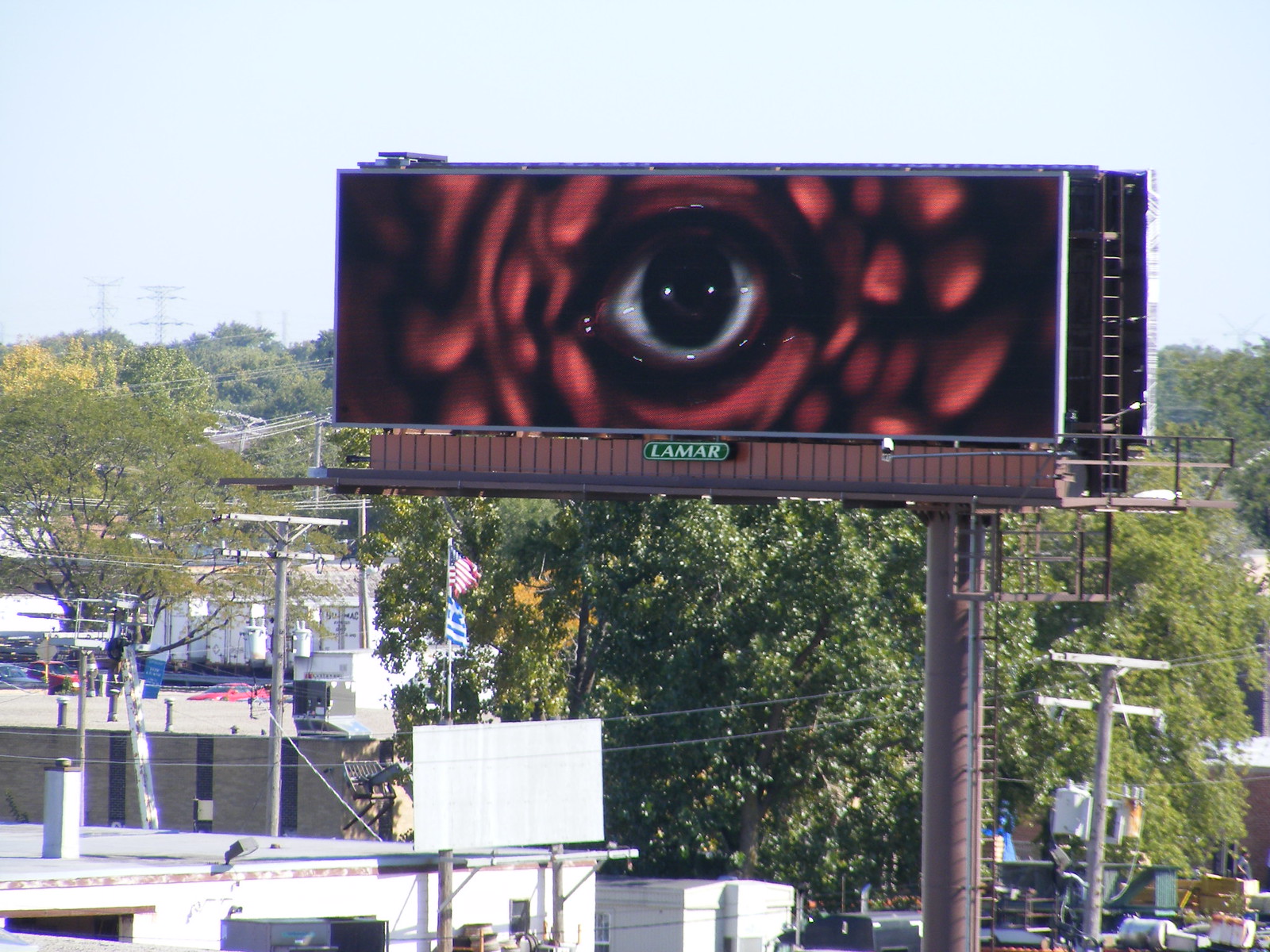This image depicts an urban billboard mounted on a large round base, positioned towards the right. The base is rust-colored and features a ladder leading up to a small platform on the right side, which has another ladder ascending to the billboard itself. The billboard appears to be digital and prominently displays a gigantic eye at its center. The eye, which looks human but evokes a dragon or demon eye, is surrounded by textured red scales or petals, possibly suggesting dragon skin or a rose. The eye is further accentuated by a white outline and a large black pupil. At the bottom of the billboard, set within a green circle, is the text "Lamar," indicating the manufacturer of the billboard. Below the billboard, power lines and utility poles are visible, and the bottom left corner shows the tops of smaller buildings. In the background, the landscape reveals hills covered with trees and prominently visible metal power lines in the top left distance, with parked cars and trees adding to the urban setting.